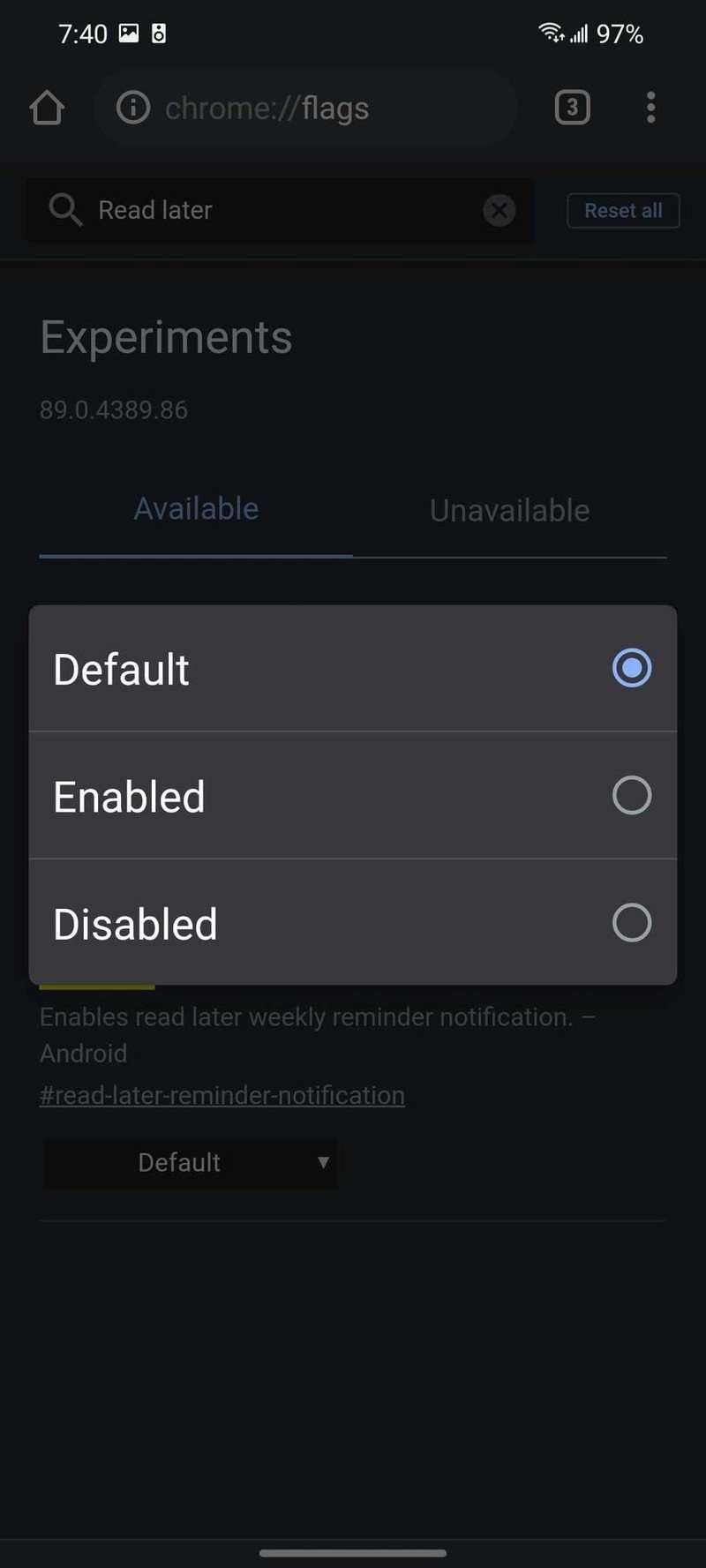The image captures a screenshot taken on an iPhone, with a 97% battery life and strong signal bars. The time displayed on the left-hand side of the status bar is 7:40. At the top of the screen, there are multiple tabs, one of which is labeled "Chrome flags." 

On the right side of the screen, there are three buttons. The first button is a house icon, indicating the home button. The second button is likely a magnifying glass icon, representing the search function, and next to it, there is an option labeled "Read Later." 

The screen is displaying a settings menu related to Chrome experimental features, labeled as "Experiments." This section is divided into "Available" and "Unavailable" options. Under the "Available" section, the selected setting is "Default," indicated by a filled blue circle, with options for "Enabled" and "Disabled" shown with unmarked circles.

Further down, there is a feature description: "Enables Read Later weekly reminder notifications for Android." Below this, the setting is again at "Default," with a dropdown menu that can be adjusted to see other options if the default setting does not suffice.